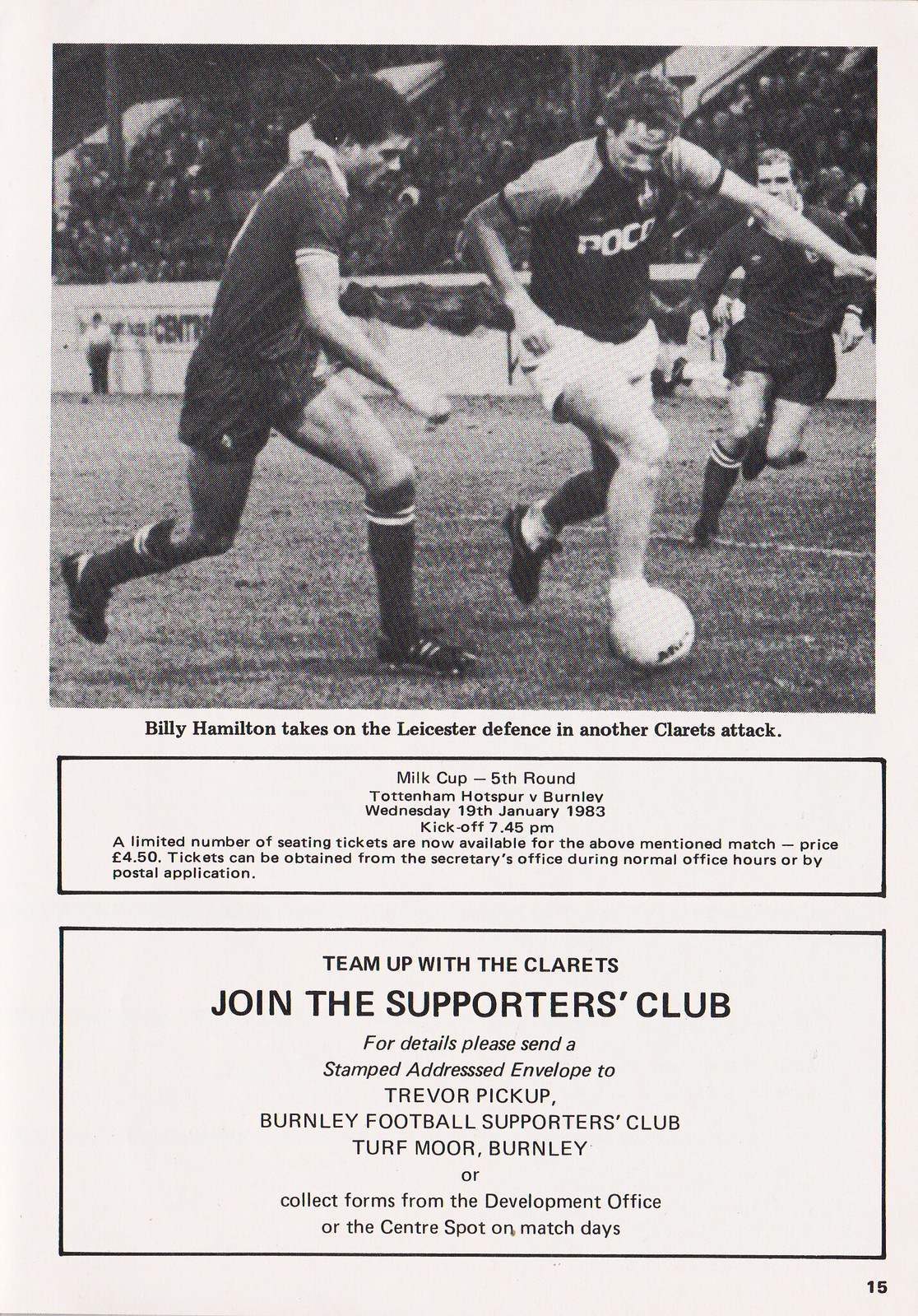This excerpt from a soccer program booklet, specifically page 15, features a striking black-and-white photograph at the top of three soccer players fiercely competing for the ball on the field, with a densely packed spectator area in the background. The caption beneath the photo highlights, "Billy Hamilton takes on the Leicester defense in another Carrick's attack." Below this image, there is a rectangular box with details about the Milk Cup 5th round match between Tottenham Hotspur and Burnley, scheduled for Wednesday, January 19, 1983, with a 7:45 PM kickoff. It mentions that a limited number of seating tickets priced at £4.50 are available, which can be obtained from the secretary's office during normal business hours or through postal application. At the very bottom of the page, another larger rectangular section encourages readers to join the Carrick Supporters Club, providing details for membership applications through a stamped addressed envelope sent to Trevor Pickup at the Burnley Football Supporters Club or by collecting forms from the development office or center spot on match days.